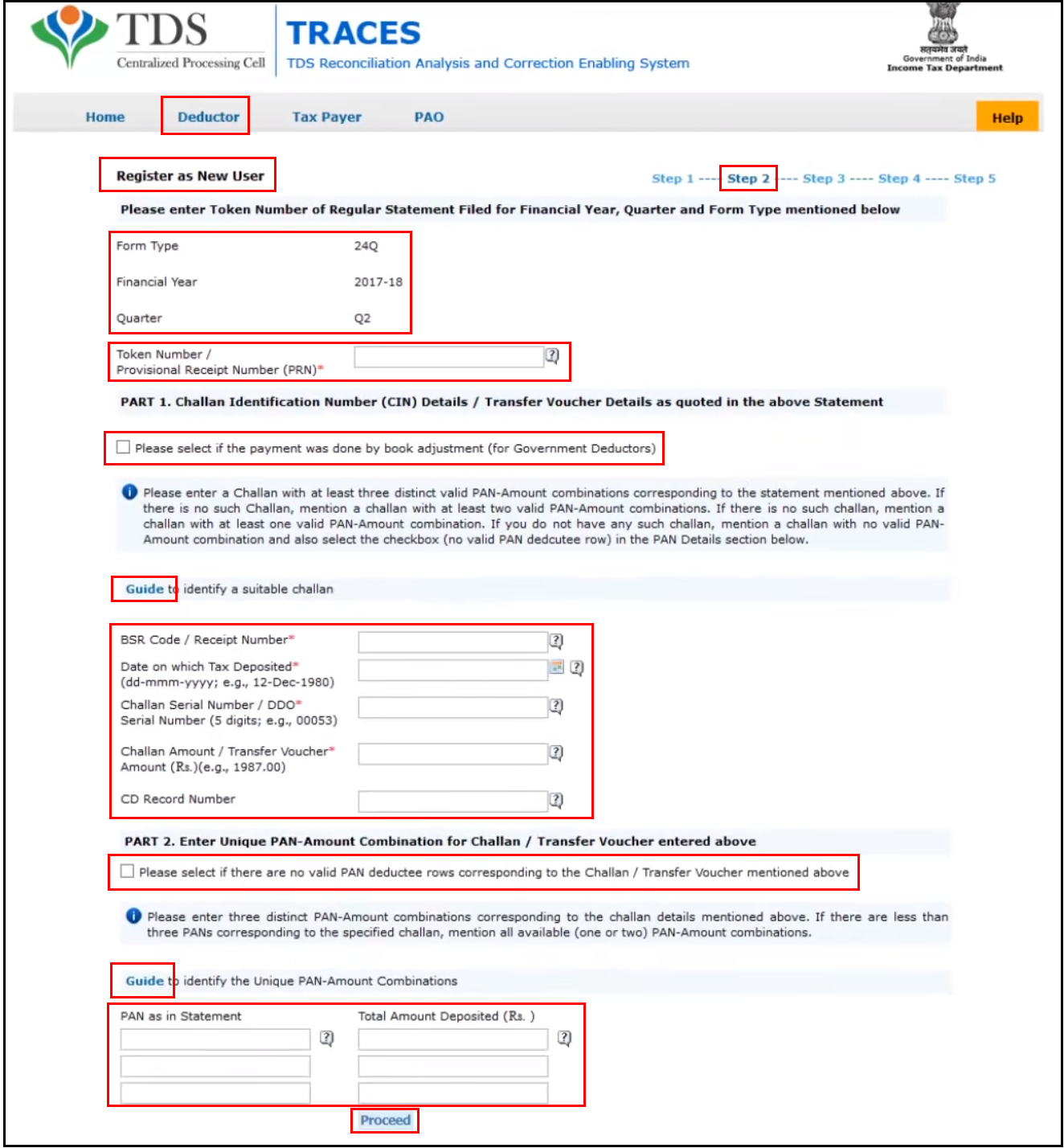The Traces TDS Reconciliation Analysis and Correction Enabling System (TDS TRACES) webpage features a series of red-highlighted boxes that denote important interactive elements. At the top of the page, navigation options include 'Home,' 'Deductor,' 'Taxpayer,' and 'PAO.' Below these, the prominent sections are detailed as follows:

1. **Deductor**: The initial highlighted box.
2. **Register as New User**: Positioned as the second interactive box.
3. **Step 2**: Located off to the side, guiding users through the next phase.
4. **Form Type**: Indicates Form 24Q for the Financial Year 2017-18, Quarter Q2.
5. **Token Number/Provisional Receipt Number (PRN)**: A field where users can input the respective numbers.
6. **Book Adjustment Indicator**: A checkmark box for government deductors to select if the payment was made via book adjustment.
7. **Guide**: Appears twice, providing additional guidance.
8. **BSR Code/Receipt Number**: An empty input field where users can enter this information.
9. **Date of Tax Deposit**: A space to fill in the deposit date in day, month, and year format.
10. **Challan Serial Number**: An empty field for entering the serial number of the challan.
11. **Challan Amount**: Another empty input field for the total deposit amount.
12. **CD Record Number**: A field to enter this number, currently blank.
13. **No Valid PAN Deductee Rows Indicator**: An optional checkmark box for instances where there are no valid PAN deductee rows in the challan or transfer voucher.
14. **PAN**: Section for entering three different PAN numbers.
15. **Total Amount Deposited**: Another section with three boxes below, all of which are currently empty.
16. **Proceed**: The final actionable button for users to move forward in the process.

This detailed description outlines each interactive element on the TDS TRACES webpage to guide users through the reconciliation and correction process efficiently.